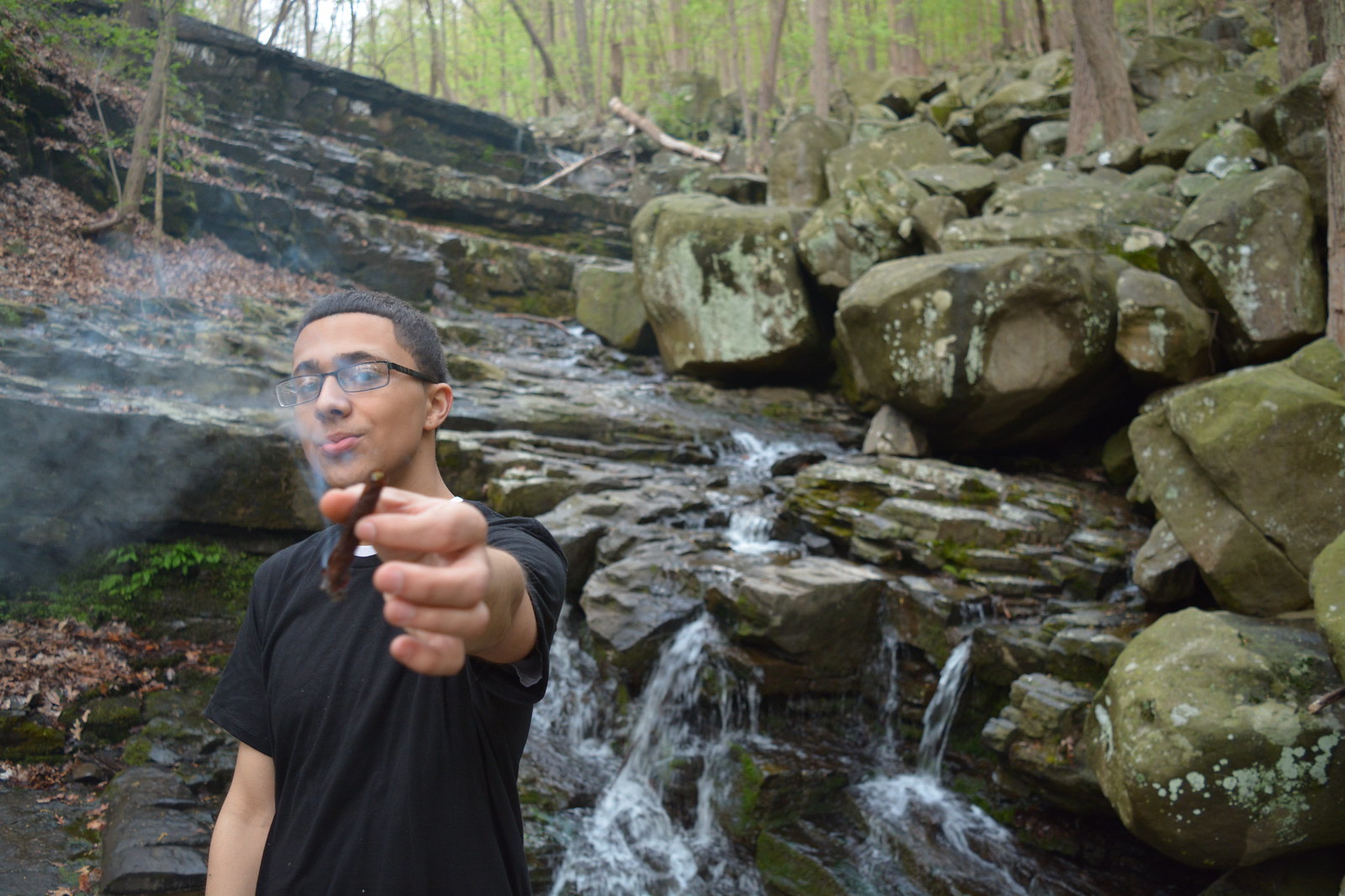A photograph captures a man standing in the lower left corner, extending his left hand toward the camera to offer a lit brown cigar, wisps of smoke curling upward. He wears a short-sleeved black T-shirt and black-rimmed reading glasses, and his youthful face has a welcoming expression. The man stands in front of a small, natural waterfall, twice his height, trickling water down a rocky hillside. The background features multiple steps of naturally formed rocks with greenery, including thin-trunked brown trees with green leaves, some dotted with moss. The sky, a light gray, peeks through the canopy, hinting it’s daytime. Surrounding the scene are boulders and undergrowth, creating the ambiance of a secluded forest trail. The water from the waterfall splashes into a creek towards the right of the man, completing this serene outdoor moment.